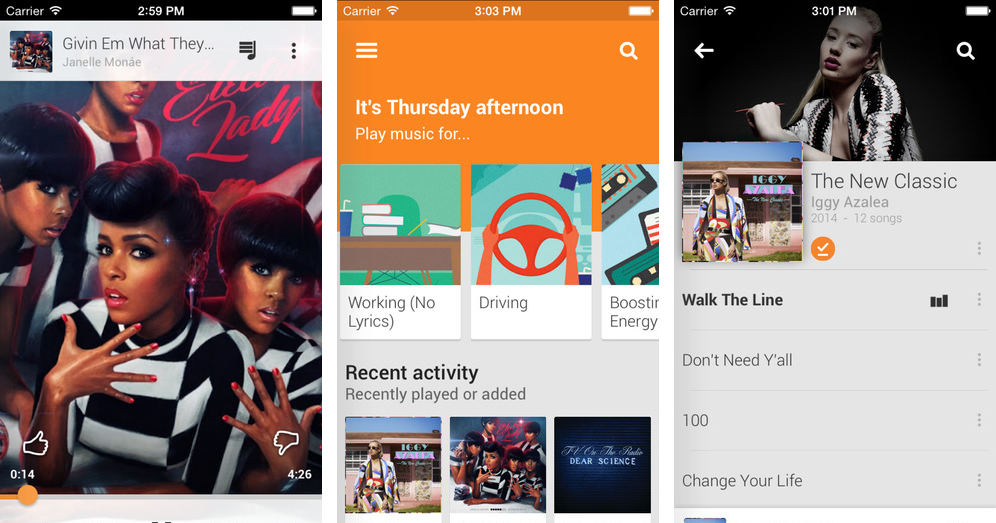In the image, on the far left side, there's a cell phone screen displaying the time as 2:59 p.m., with a full battery icon in white. The phone screen shows a music player with the song "Give Them What They Want" by Janelle Monáe. Below the track name are several women, all dressed in black and white striped tops, with pink-painted nails, holding their hands out in front of them.

In the center of the image, there's a vertical orange rectangle with the time displayed as 3:03 p.m. The background has an orange and white color scheme with text that reads, "It's Thursday afternoon, play music for..." followed by options such as "working (no lyrics)" and "driving." Underneath this section, there's a "Recent Activity" list showing albums from Iggy Azalea and Janelle Monáe. The last album in the list has a navy blue background and is titled "Bare Science."

Finally, another cell phone screen shows the time at 3:01 p.m., with Iggy Azalea's album "The New Classic" displayed. Behind her, the background is black, with details indicating the album was released in 2014 and contains 12 songs. The current track being played is "Walk the Line," followed by "Don't Need Y'all," "100," and "Change Your Life."